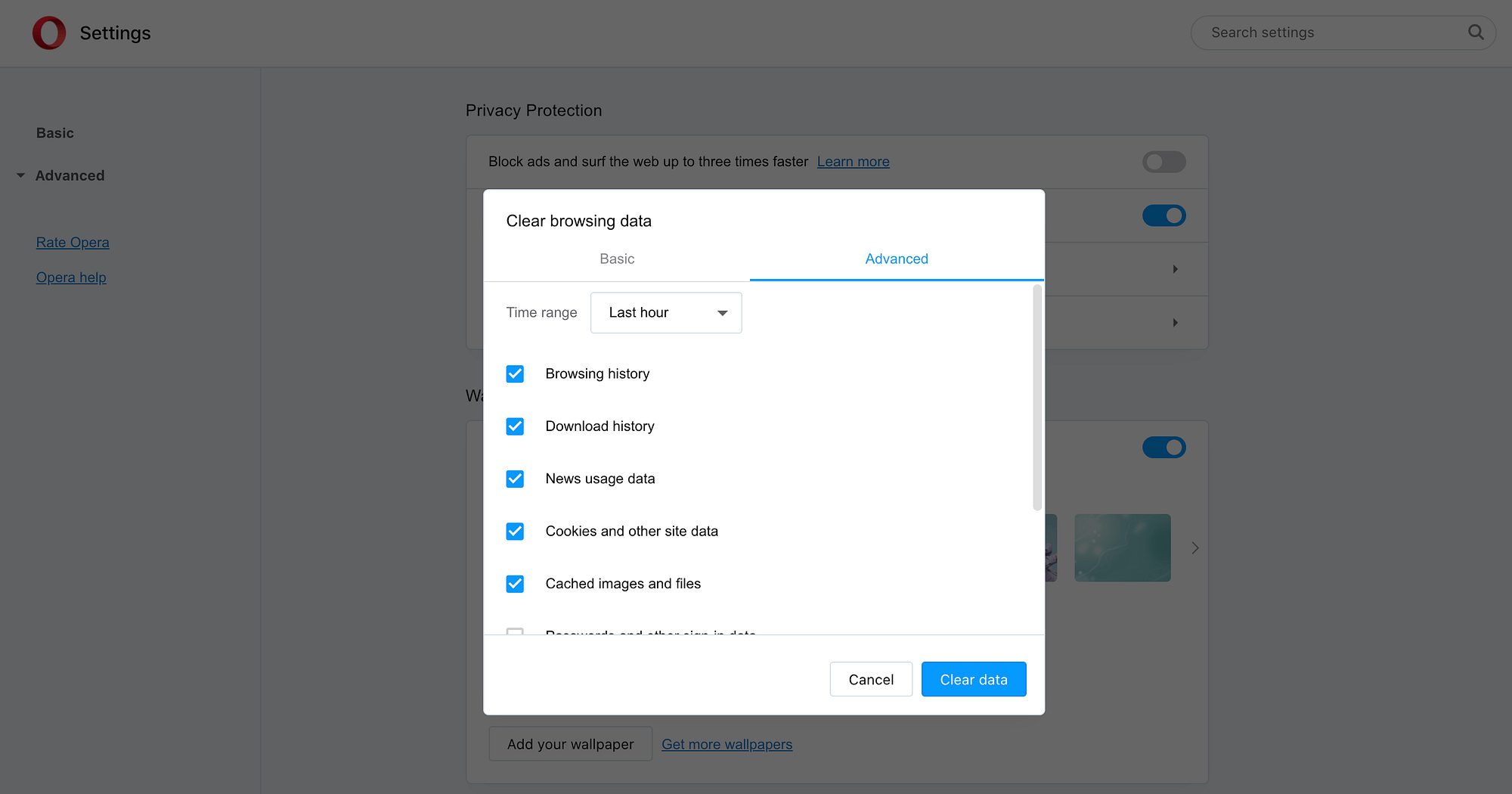Screenshot of Browser Settings Interface

The image captures a screenshot of a browser's settings interface, highlighting the "Privacy Protection" section. In the foreground, there is a prominent red circle, possibly indicating a notification or error. The central focus is a white pop-up window titled "Clear Browsing Data," set to the "Basic" tab. It offers options to clear data within a specific "Time range," currently set to "Last hour." Below, checkboxes are available for various types of data: "Browsing history," "Download history," "Cookies," and "Cached images." A blue button labeled "Clear data" is prominently displayed at the bottom of the pop-up. In the background, glimpses of the main settings interface are visible, showing options for "Advanced" settings and additional customization, such as changing the wallpaper.